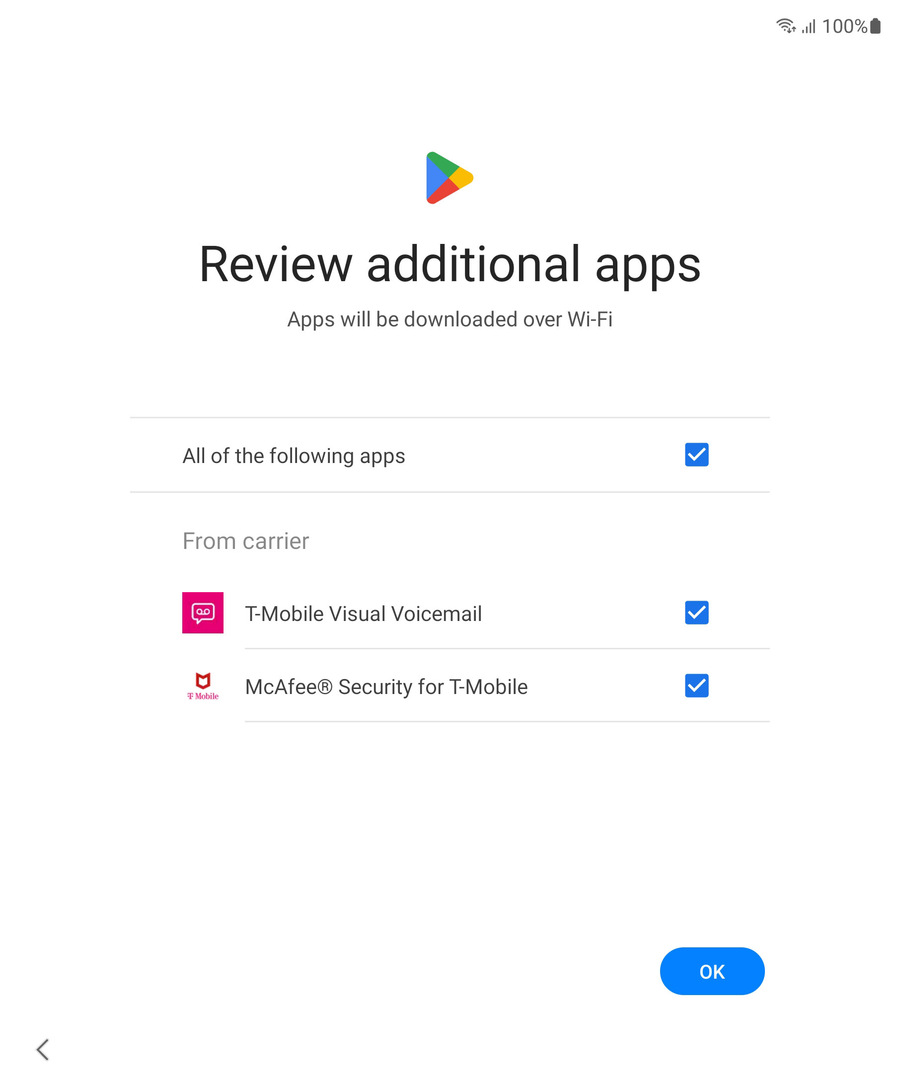This is a screenshot captured from a cell phone, where the battery is fully charged at 100%, as indicated in the upper right corner. The screenshot is set against a completely white background. Prominently centered at the top is the Google Play logo, noted for its multicolored arrow featuring shades of blue, red, yellow, and green. Below this logo, a message reads: "Review additional apps. Apps will be downloaded over Wi-Fi."

Underneath the message are three checkboxes aligned vertically on the right side, all of which are selected and marked with a blue background and a white checkmark. The first checkbox on the left corresponds to the option labeled "All of the following apps." Below this, two more options are listed: "From carrier," which is not a clickable option but rather a heading. The subsequent checkboxes are for "T-Mobile Visual Voicemail" and "McAfee Security for T-Mobile," both of which are also checked.

In the bottom right corner of the screenshot, there is a prominent blue button labeled "OK," which is intended for confirming the selected apps. The image details the selection of carrier-specific apps that will be downloaded over Wi-Fi, specifically T-Mobile Visual Voicemail and McAfee Security for T-Mobile.